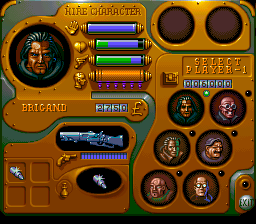This is a detailed descriptive caption for the image:

"The screenshot captures a moment from a rudimentary video game, presented in a square format. The game interface features a predominantly green background with gold accents. At the top of the screen, the text 'H-I-R-E' signals the option to hire a character. Below this, a circular portrait of a character's head is displayed, accompanied by three horizontal progress bars with fluorescent lighting: these bars are blue or green, indicating varying levels of specific characteristics such as health, stamina, or power.

On the right side of the screen, two empty character circles are visible, suggesting available slots for additional players or team members. Below these, six circles contain headshots of other available characters, offering options for selection. Just above these character portraits, the text 'SELECT PLAYER 1' designates the prompt for choosing the primary player. The current score reads '006000,' hinting at the player's progress.

In the bottom-left corner, the character's ammunition inventory is detailed, showcasing icons for a shotgun, bullets, a handheld gun, and a corresponding progress bar indicating available ammo. This screenshot encapsulates the game's core elements such as character selection, health and ammo statuses, and functional gameplay metrics in a nostalgic, primitive gaming aesthetic."